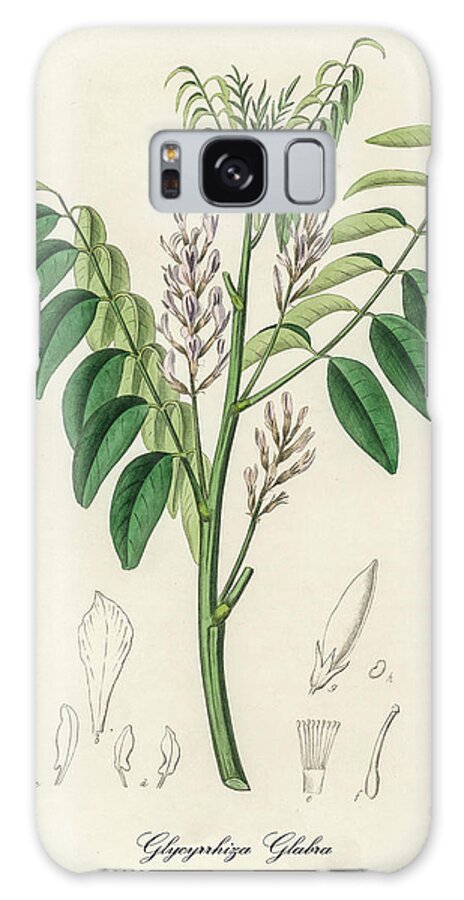The image showcases the back of a cell phone adorned with a protective case. The case is primarily white with a subtle milkiness to it, highlighting an intricate and artistic botanical design. Dominating the pattern is a green plant featuring a single main stem with two smaller branches bearing various shades of green leaves. Interspersed among the leaves are tiny, light purple flowers and brown grains, possibly seeds, adding a touch of earthiness to the design.

In the lower portion of the case, delicate, pencil-like botanical sketches of different leaves add an artistic and unfinished feel to the botanical motif. Below these sketches, an elegant cursive inscription can be found, written in black ink, which appears to spell out "GLYCAPRHIZAGLABRA" in a foreign, sophisticated script.

At the top center of the phone's back, the camera module is situated, housed in a rectangular gray area. The module itself is a black square, flanked by additional rectangular features, including the flash and fingerprint sensor, adding to the phone's functionality while minimally disrupting the artistic design of the case.